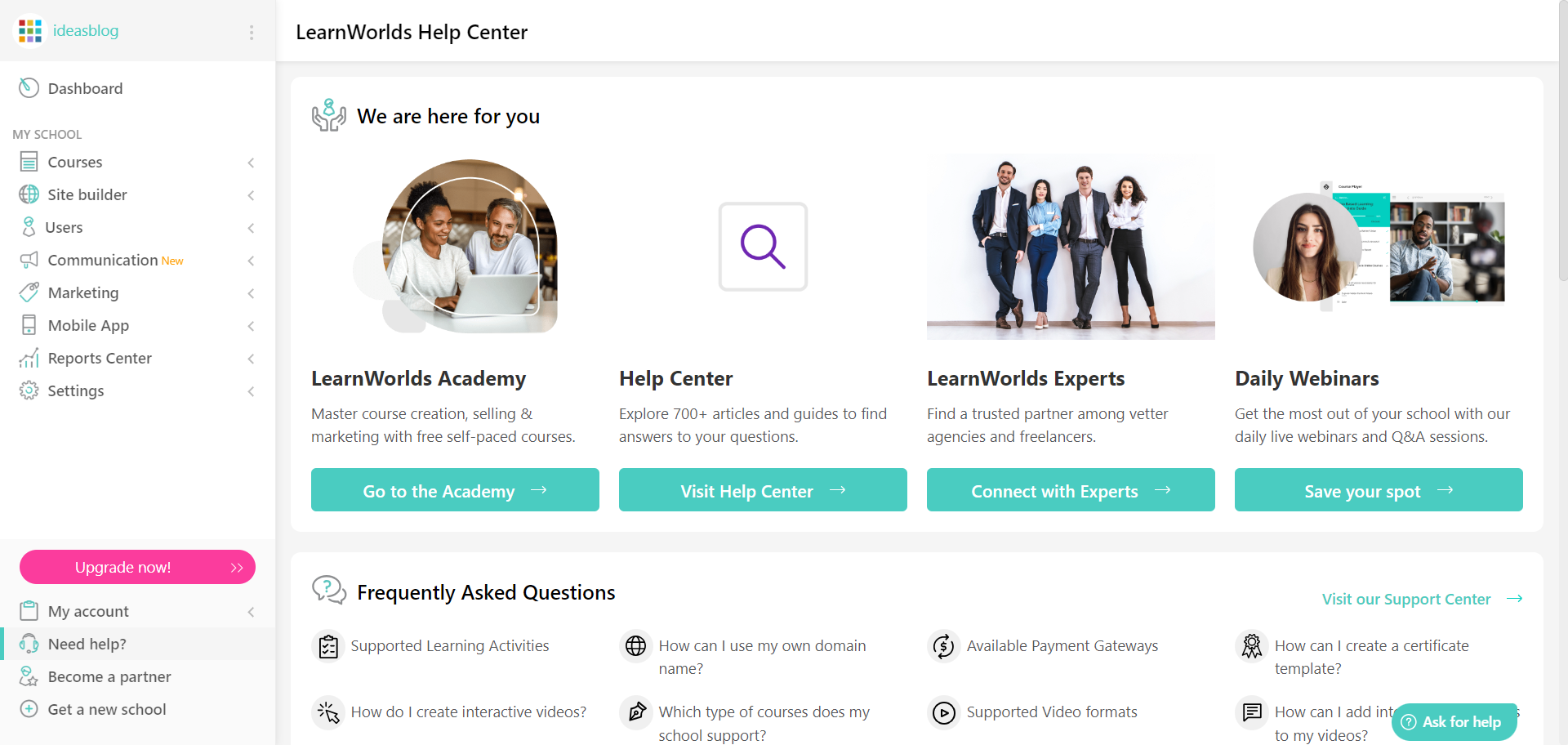**Caption:**

The image is a detailed screen capture of a blog site interface, identified in the upper left corner as "Idea Blog." To the left, a vertical navigation column lists various dashboard options: My School, Courses, Site Builder, User Communications, Marketing, Mobile App, Report Center, and Settings. Beneath these options, there are additional links: Update Now, My Account, Need Help, Become a Partner, and Get a New School.

Dominating the right side of the screen, the header "LearnWorld's Help Center" welcomes users with a message, "We are here for you.” Below this header are four horizontally aligned information blocks: LearnWorld Academy, Help Center, LearnWorld's Experts, and Daily Webinars.

At the bottom of this section, an FAQ area is visible, covering topics like support, learning activities, and creating interactive videos. The primary focus of the interface is the help center, offering quick access links such as Go to the Academy, Visit Help Center, Connect with Experts, and Save Your Progress.